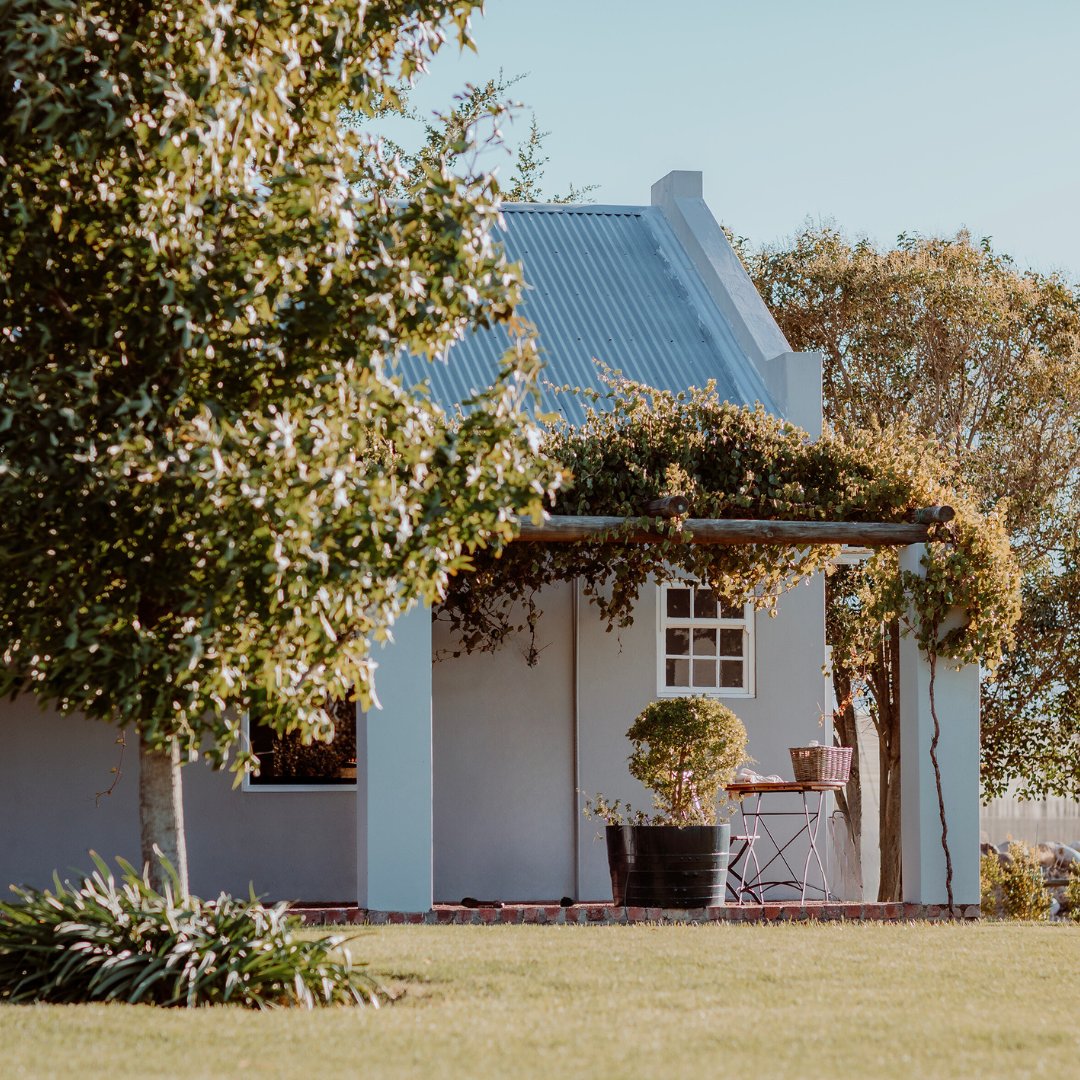This image captures the exterior of a simple, single-story house with stucco walls and a corrugated metal roof. The house features a small front porch supported by two white pillars, with a wooden beam structure covered in green ivy draping down onto the pillars. On the brick patio below, there is a cozy seating area with a chair and a slim table, which holds a picnic basket. In front of the seating setup is a large black planter containing a small tree. The yard is mostly green, although the grass is somewhat patchy and tan. Two windows with white frames are visible, and the sky is a clear blue. To the left of the house is a large, leafy tree with a smaller green plant at its base, partially obscuring the view of the home. Trees also frame the scene on both sides, enhancing the garden-like atmosphere of this charming outdoor space.